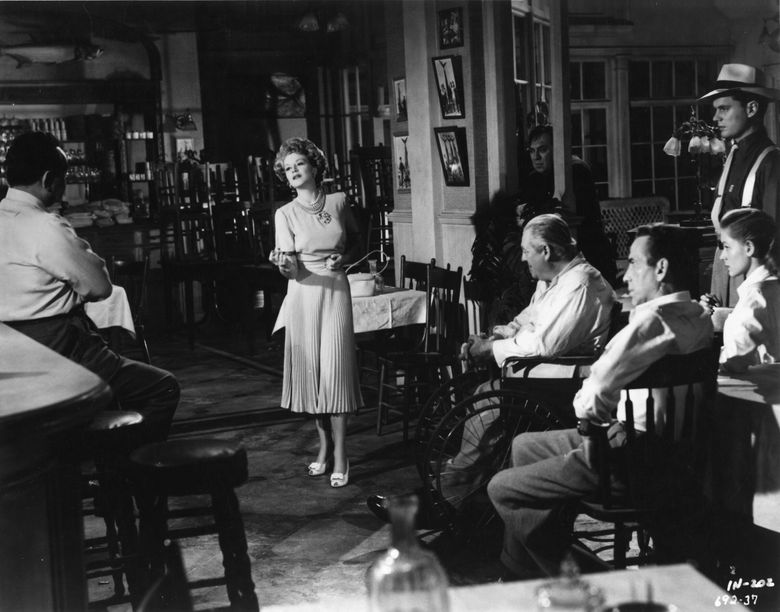This black-and-white vintage photograph, likely taken between the 1940s and 1960s, depicts an interior setting of a bar at night. Central in the image is a woman wearing a white pleated dress, high heels, and makeup with curled hair and jewelry, striking a pose with her right arm stretched out, suggesting she might be dancing or performing. Surrounding her are seven individuals, primarily men, all seemingly focused on her. To the left, one man is seated on a bar stool, and to the right, another man in a fedora or cowboy hat stands alongside two other men and a woman who are seated. One of the seated figures appears to be in a vintage wheelchair. The patrons, who have neutral expressions, are mostly attired in white or dark shirts with dark slacks. Details such as bottles of wine on tables and pictures on the walls contribute to the setting. The bar’s ambiance appears closed or after-hours, indicated by chairs propped on tables.